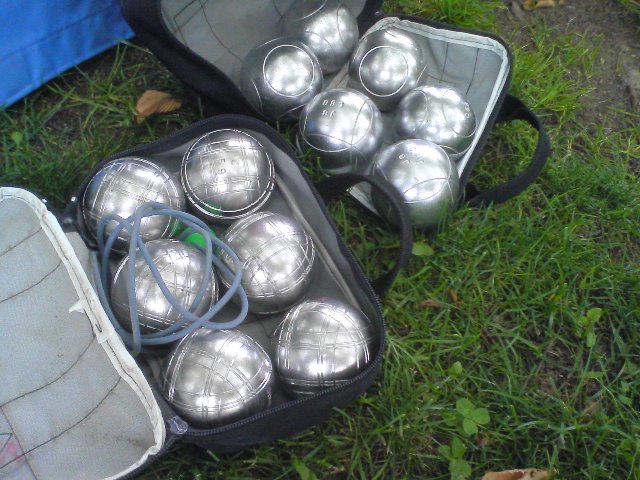The image shows two black bags with black handles resting on green grass, likely indicating a springtime setting. Despite the vibrant grass, the day appears overcast with no direct sunlight visible. Each bag is black on the outside and grayish silver on the inside, with lighter grayish silver trim. Both bags contain six silver metal balls with intricate line designs. One notable feature in the first bag is a blue rope laying atop the second silver ball. Additionally, the bottom right corner of the image contains small shamrock plants, and the upper right shows some exposed dark gray dirt. In the upper left corner, a small piece of a blue object is partially visible, though its identity is unclear.